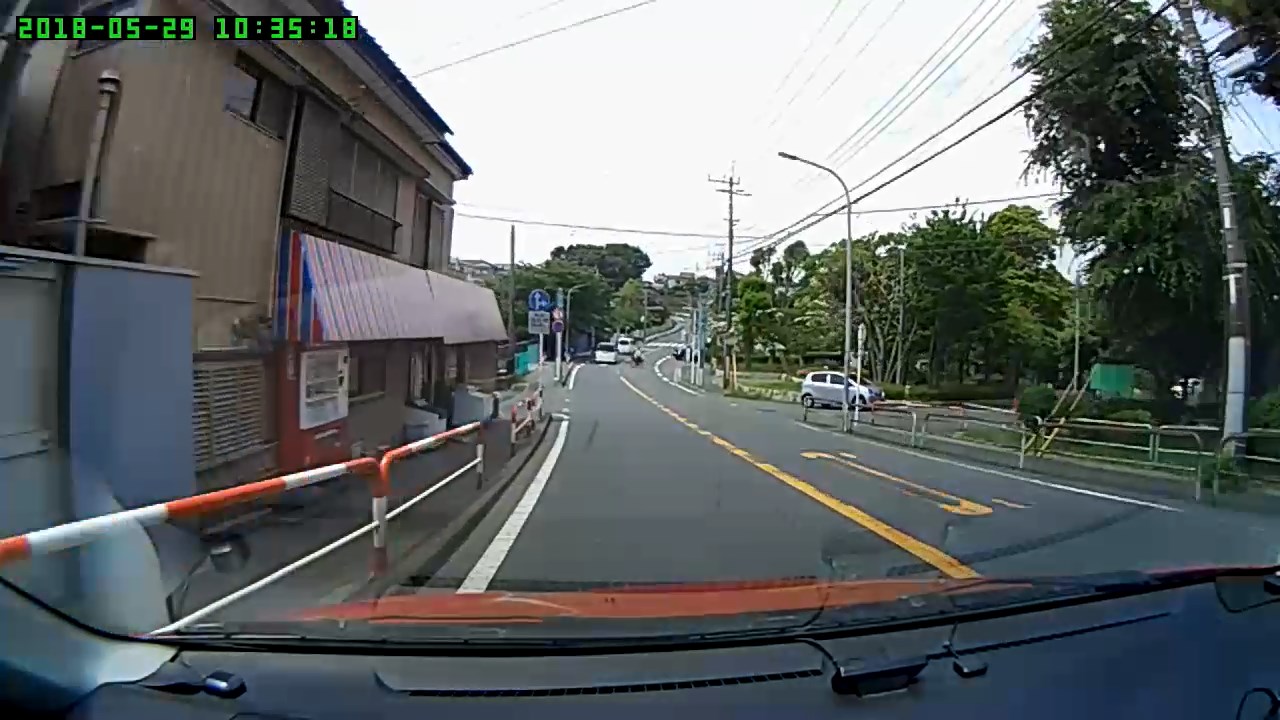This color photograph, taken during the day from inside a vehicle, offers a view through the windshield down a street. On the left side, a building lines the street, bordered by a sidewalk separated from the road by hand railings. In the distance, a couple of buses can be seen approaching from behind. On the right, a motorcycle or bicycle travels in the opposite direction. The right side of the image also features a variety of greenery, a parked car, numerous trees, and telephone poles adorned with wires extending along the street. The sky appears almost white, giving a bright and overcast ambiance. The date "May 29, 2018" and the time "10:35:18" are prominently displayed at the top of the image.